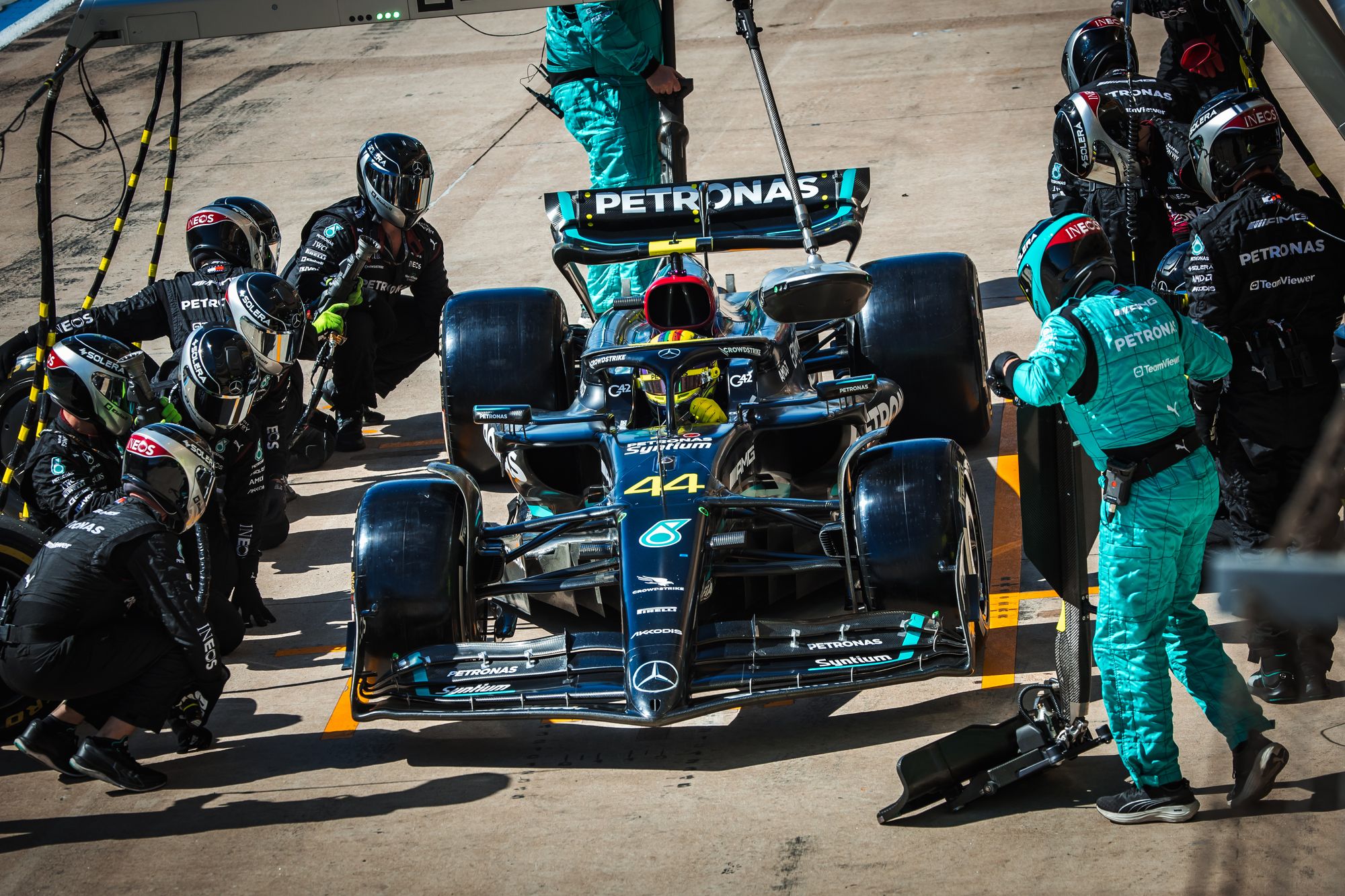In the center of the image, an imposing black Formula One car with steel accents and the number 44 prominently displayed on its front stands poised for action. The F1 car, marked by its sleek design and emblazoned with "Petronas" in white letters on the rear wing, features a driver sporting a striking red helmet with a black visor, glimpsed through the car's open cockpit. Surrounding the vehicle, a meticulously coordinated crew is positioned: on the left side, five crew members in standard racing jumpsuits and helmets are crouched attentively, while on the right, a line of standing crew members mirror their vigilance, all uniformly attired in Petronas-branded gear with black and teal accents. The crew's precise arrangement and focused stances suggest a critical pre-race check or a rapid pit stop, taking place on a light tan racetrack marked by black smudges and a defining yellow pinstripe. The image captures the intense preparations and synchronized efforts central to Formula One racing.